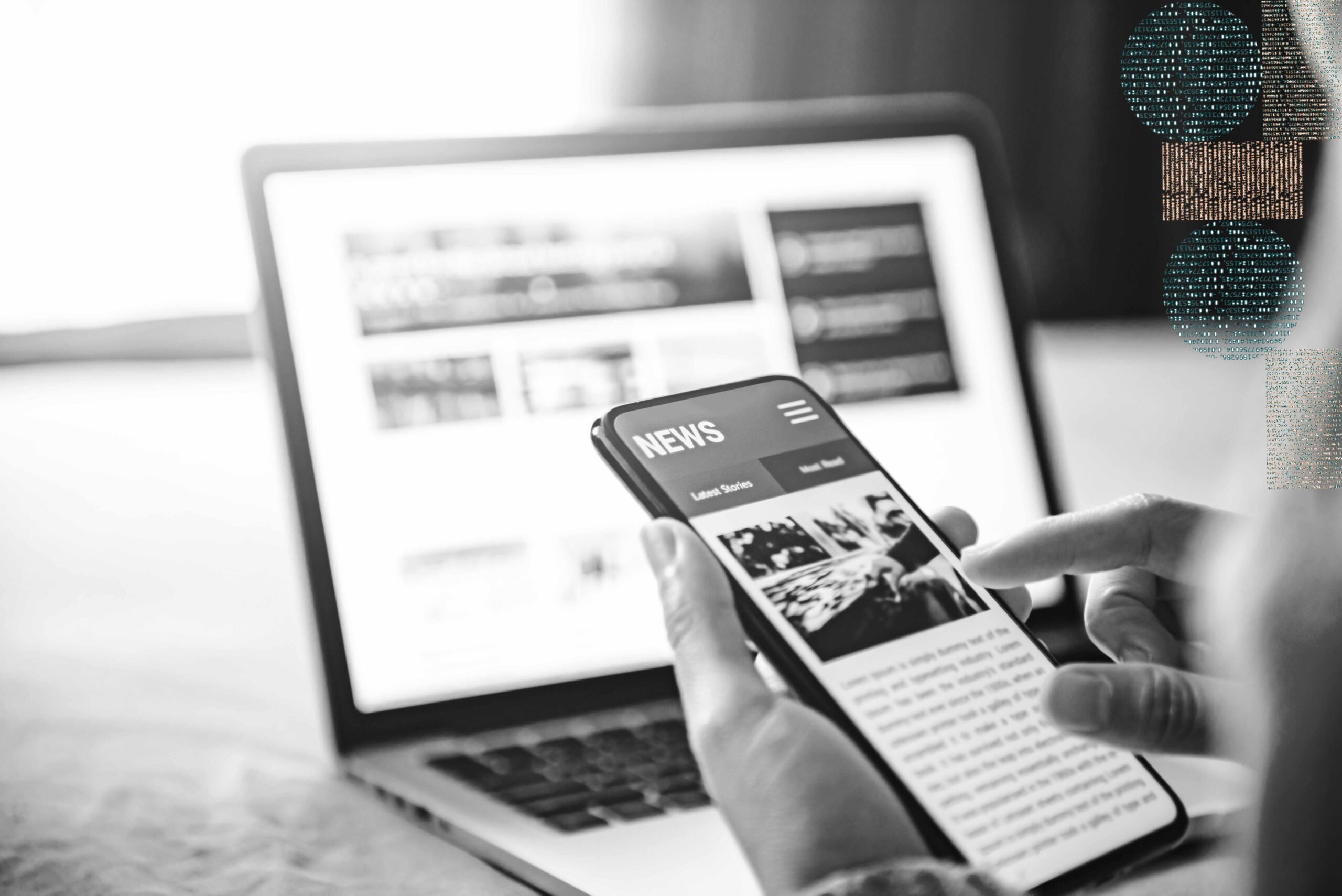In this black and white photograph, the focal point is a slightly out-of-focus laptop positioned centrally on a blurred surface, suggesting a serene indoor setting. Bright white sunlight streams through a window in the upper left corner, casting a natural glow over the scene. In the foreground, we clearly see a pair of hands engaged with a smartphone. The left hand holds the device, and the right hand appears to be scrolling through a news article, which is faint but visible under the "News" header at the top left of the phone screen. The scene conveys an introspective moment of browsing the news in a tranquil environment. Notably, in the upper right corner of the image, abstract shapes consisting of two blue circles and several semi-translucent beige and pink rectangles contribute to the artistic quality of the photograph.